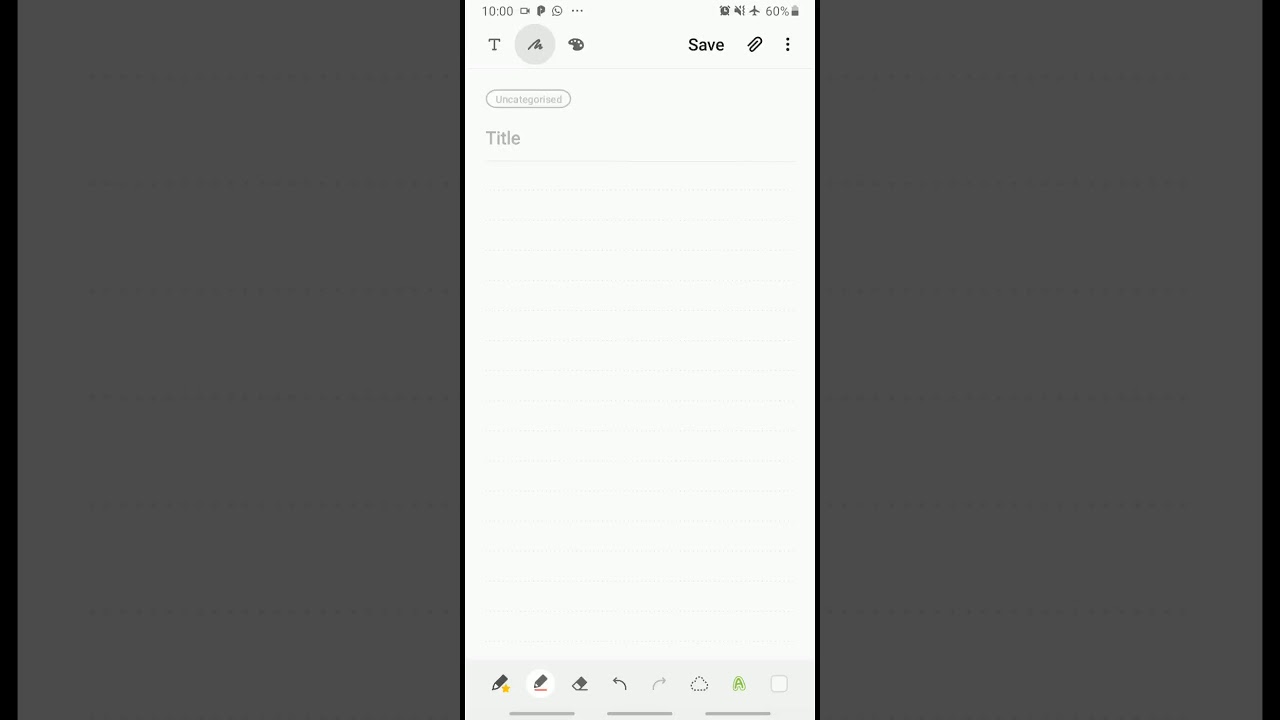In the image, there is a detailed screenshot of a smartphone screen at exactly 10:00. 

At the top left corner, the time is displayed alongside several icons: a camera symbol, a "P" symbol, a clock symbol enclosed in a circle, and three vertical dots. Moving to the top right corner, additional icons can be seen: an airplane mode indicator, another clock symbol, and an unspecified icon. Further to the right, the battery percentage and battery icon are shown.

The center top portion of the screen is blank, creating a clean division between the icons above and the content below. Directly beneath the time display, there's a letter "T" followed by a scribble encased in a gray circle. Adjacent to this, on the right-hand side, is a symbol resembling a painter's palette. Below this icon, closer to the battery area, the word "SAVE" is prominently displayed, accompanied by a paperclip symbol and three vertically aligned black dots.

Beneath this cluster of symbols, the word "Uncategorized" appears in gray, followed by the word "Title." The rest of the screen remains white and blank, providing a stark contrast to the top features. At the bottom of the screen, additional functional icons are visible, including a back arrow, suggesting navigation options.

Overall, the image captures a complex yet organized layout of a smartphone screen, focusing on the array of icons and functionalities presented in a user interface.